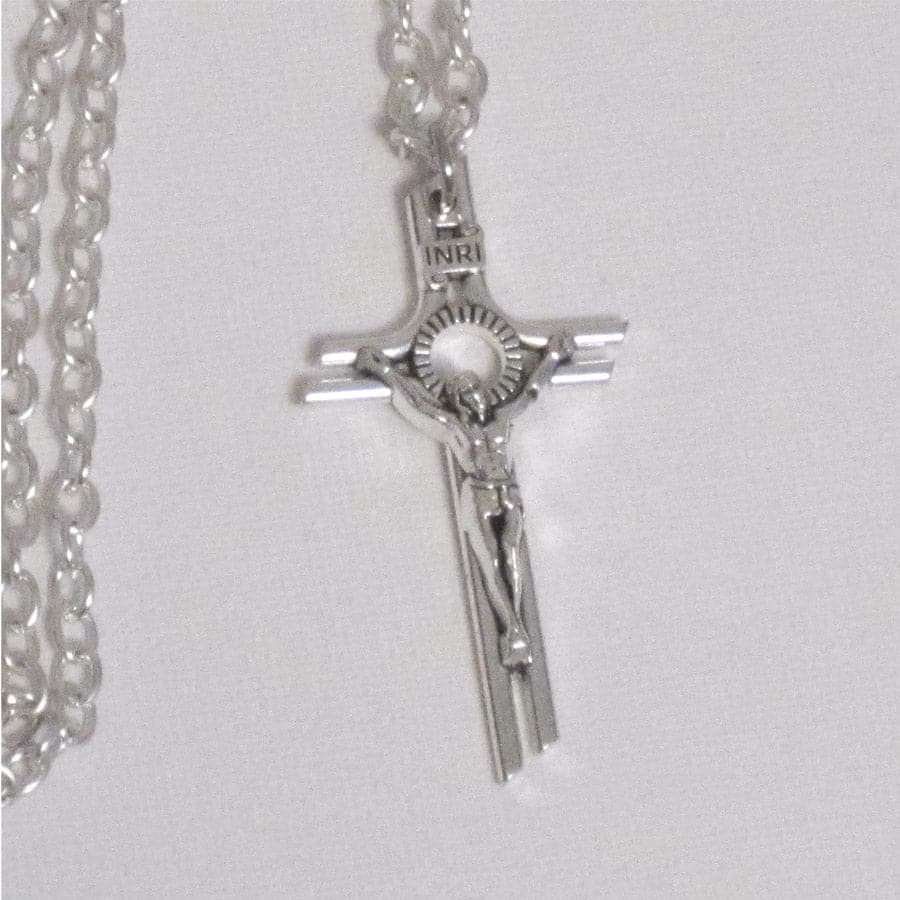This black-and-white photograph captures a detailed view of a silver crucifix necklace prominently placed at the center of the image. The crucifix, featuring an intricately designed Jesus with arms outstretched along the crossbar and legs together along the vertical pole, is affixed to a chain. Above Jesus' head, the initials "INRI" are inscribed, referencing the Latin phrase “Iesus Nazarenus, Rex Iudaeorum” (Jesus the Nazarene, King of the Jews). A ribbed halo frames Jesus’ head, which is slightly tilted towards his right arm. The crucifix itself appears to consist of interconnected segments forming the traditional cross shape. The necklace rests against a textured white surface, which resembles a pitted cloth or linen. The black-and-white color scheme enhances the grayscale contrasts, spotlighting the silver tones of the crucifix against the light background. The entire composition draws focus to the detailed craftsmanship of the crucifix and the serene repose of Jesus depicted on it.